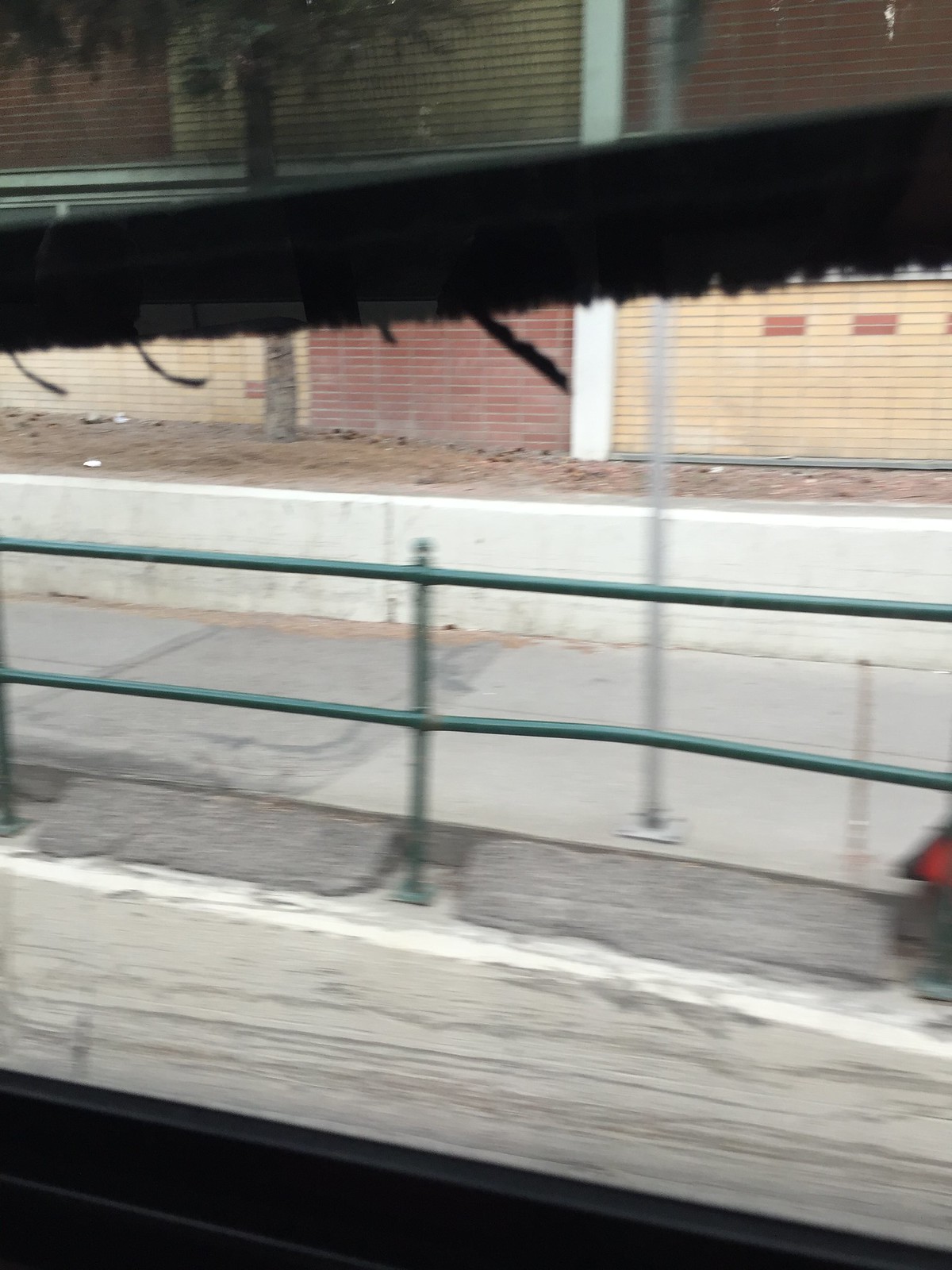The image captures an outdoor scene viewed from inside a moving vehicle through an open window. The upper part of the frame includes the top of the car window, partially obscured by drawn black blinds, and a clean windowsill. The photo is slightly blurry but still clear enough to make out the details. In the foreground, there is a green metal railing with horizontal beams, mounted on a white cement block, that stretches horizontally across the image. Just beyond the railing, there is a steep drop of about three feet down to a cement road. Adjacent to this drop, a set of dirt and a tree are visible. In the background stands a red and cream (or possibly red and yellow) colored brick wall composed of small rectangular bricks. The photo is taken during what appears to be daylight hours, adding a natural brightness despite the darker silhouette of the car window at the top. No people or text are present in the image.